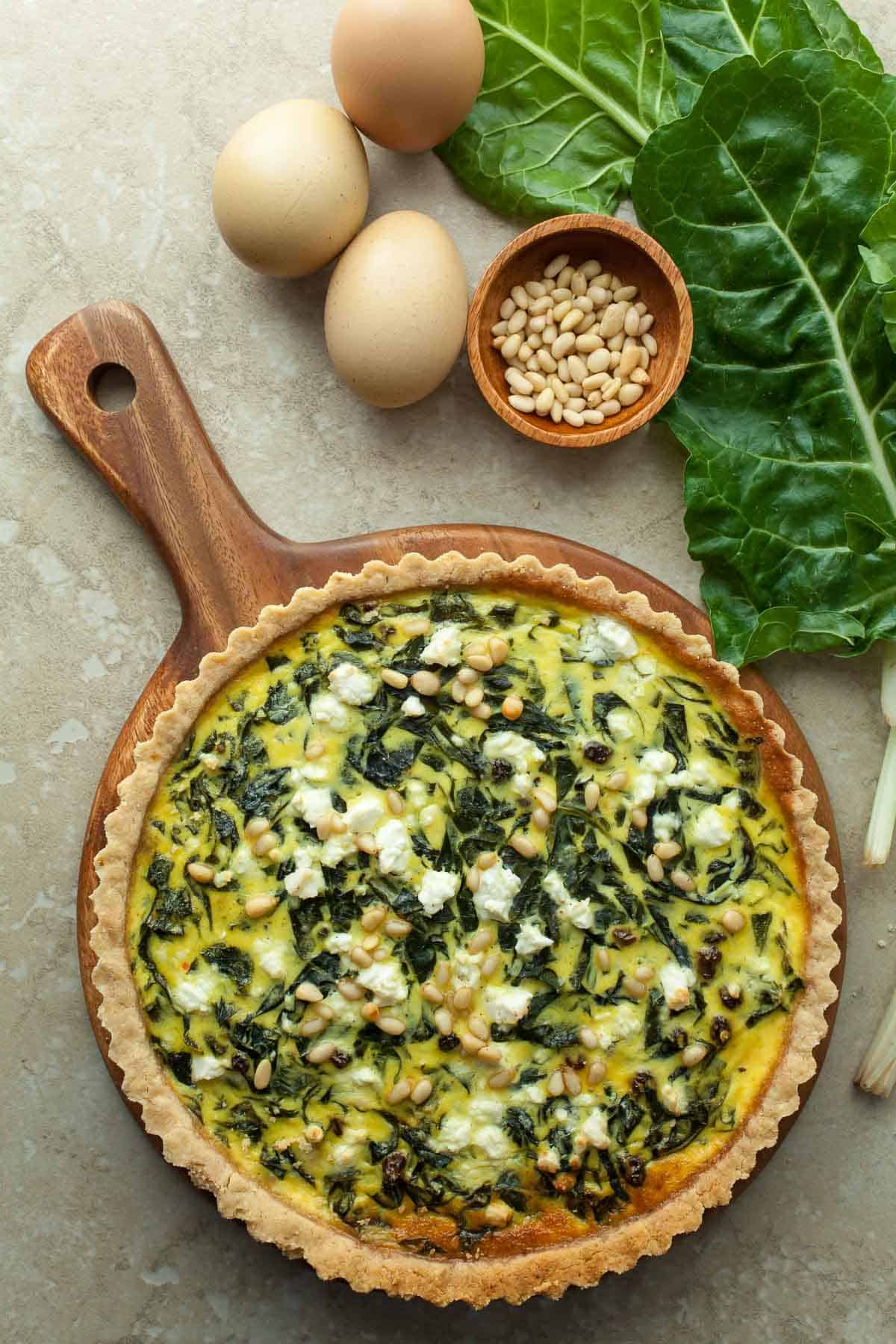This image presents a close-up view of a meal centered around a pie, captured from above. The pie, which appears to be placed on or in a light brown wooden kitchen piece with a handle and a hole at its end, displays a light brown crust that is slightly burned on the bottom and top right, yet overall looks well cooked or possibly underdone. The pie seems to contain a mixture of ingredients including spinach leaves, pieces of feta cheese, and a potentially cheesy or creamy yellow-orange substance. 

In the top section of the image, just left of the center, there are three brown eggs, two of which are light brown and one a darker shade. Between the eggs and a cluster of dark green spinach leaves in the upper right corner, a small wooden bowl sits filled with small, tan bean-like objects, which resemble light brown peas or seeds. All these elements are arranged on what appears to be a gray marble countertop, adding a contrasting backdrop to this appetizing composition.